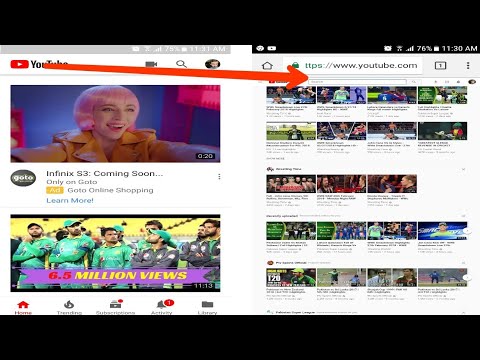Here is a detailed and cleaned-up caption for the image:

---

The image is a busy composite screen featuring two distinct sections. On the left side, there's an announcement for the Infinix S3, stating "Infinix S3 coming soon only on go to go to online shopping learn more," followed by "6.5 million views." This text is superimposed over a screenshot of a video showing several men in what appears to be a racing team, identifiable by their uniforms. 

On the right side, another screenshot from YouTube shows a grid of 19 different video thumbnails, each with unreadable descriptions beneath them due to the small size. The status bar at the top of the screen displays a 76% battery level and the device's time, indicating it's taken from a cellphone. These thumbnails depict various individuals engaging in different sports and activities.

---

This caption combines and refines all elements described, providing a clear, detailed overview of the image.